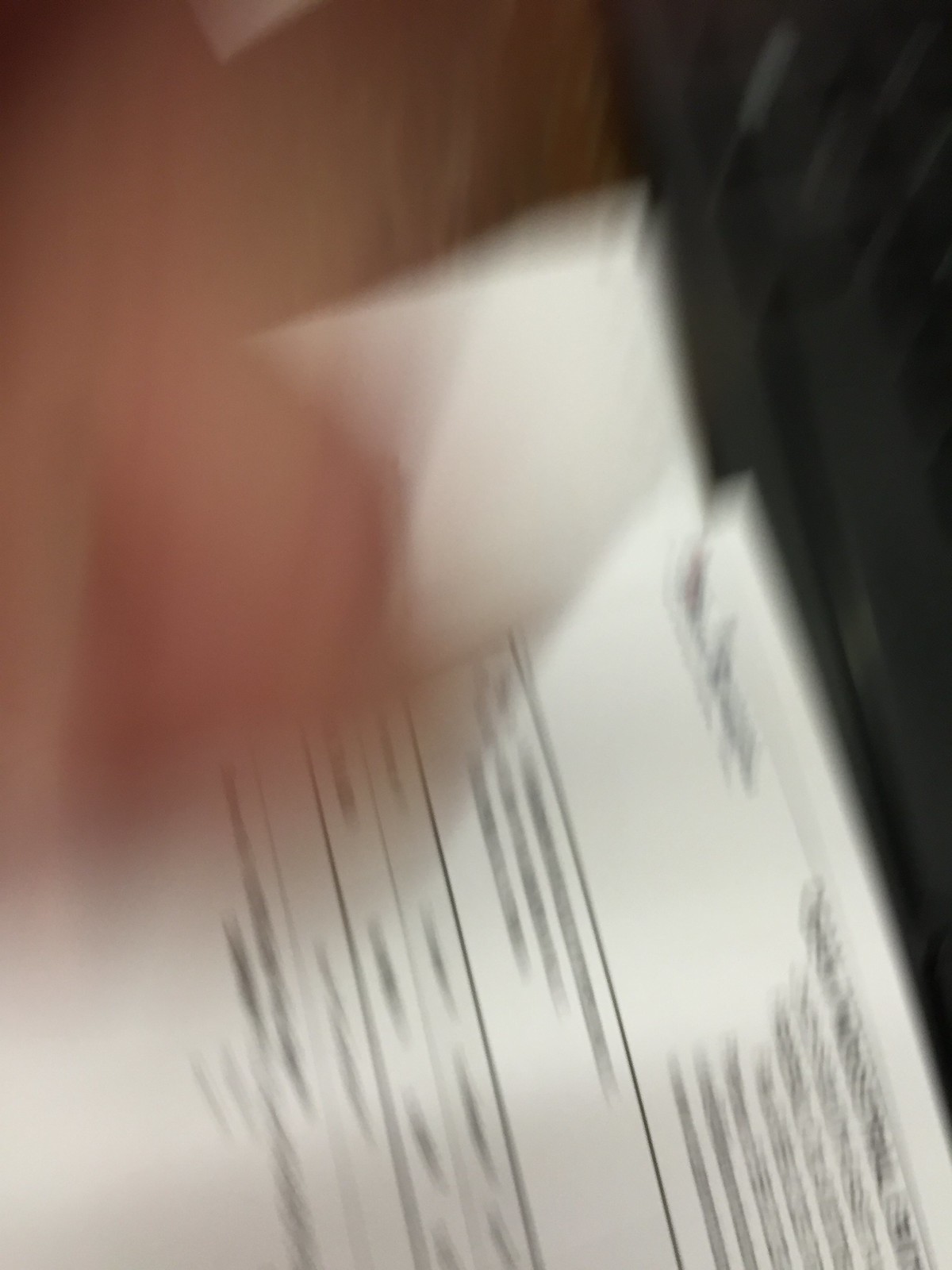A heavily blurred photograph featuring a finger intruding from the left side. The background includes a mix of dark and brown hues on the right and left, respectively. At the center, a slightly illuminated piece of white paper, appearing to be in the process of being folded, is visible. The paper bears black text and rectangular shapes, indicative of an invoice or some document, but the text is not clearly legible. The overall image is quite indistinct, making it difficult to discern finer details.